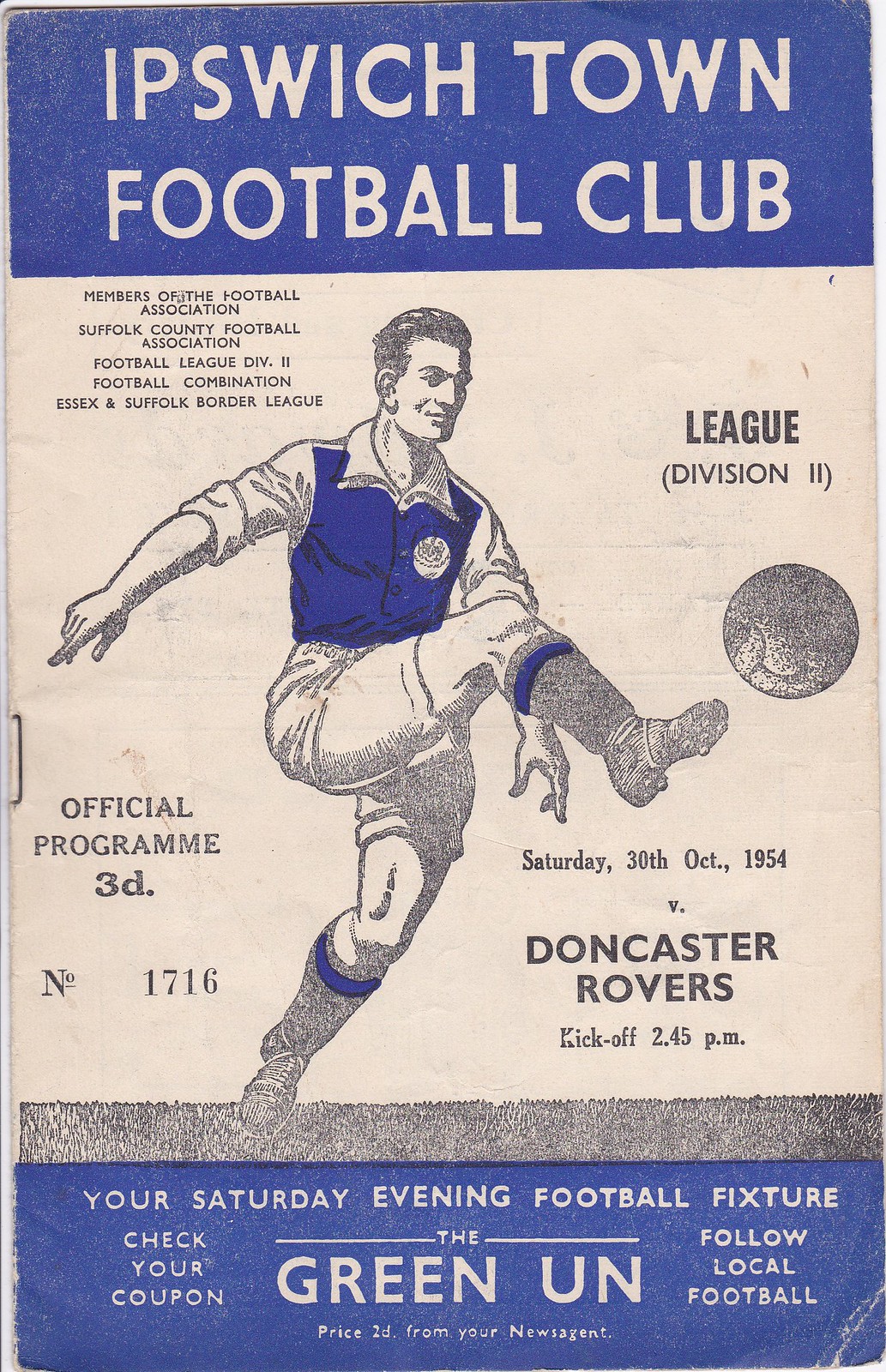The image showcases an old promotional document for a soccer game organized by the Ipswich Town Football Club. The layout prominently features blue bands with white text at the top and bottom. The top band reads "Ipswich Town Football Club," while the bottom band includes various details such as "Doncaster Rovers," "Kickoff 2.45pm," and mentions of an official program priced at 3D. The poster also references "League Division 2," "Football Association," "Suffolk County Football Association," and other associations, with some text slightly blurred. At the center of the document, set against a white background, there is an artistic monochromatic rendering of a man in a blue jersey, white shorts, and grayish socks, kicking a soccer ball with his right leg while his left leg remains grounded. The man is depicted with short hair and a smile on his face. Additional text on the poster specifies the date as "Saturday 30th October 1954" and notes it is the "Official Program, Number 1716." The lower section of the document also mentions "your Saturday evening football fixture, the Green UN."